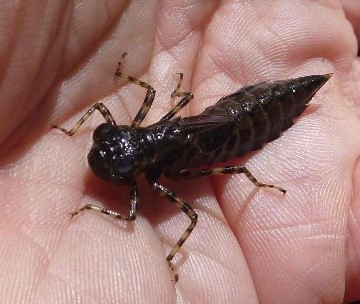This close-up photograph captures an insect cradled in the palm of a white person's hand. The image is highly detailed, focusing on the small, dark brown creature which is nearing black in color. The insect, not yet fully grown, possibly in its nymphal stage, has a cylindrical body that tapers to a pointed end, resembling a stinger. The lower half of its segmented abdomen is adorned with ridges that create a ringed look. It has six legs, three on each side of its body, which are black and yellow. The legs extend from just behind the head and continue down to the bottom of the thorax, ending before the ringed abdomen. The insect's head is slightly darker than its body, and its eyes are clearly visible, giving an impression that the bug might be looking up at the photographer. While uncertain of the exact species, the detailed attributes hint it could potentially mature into a cicada.